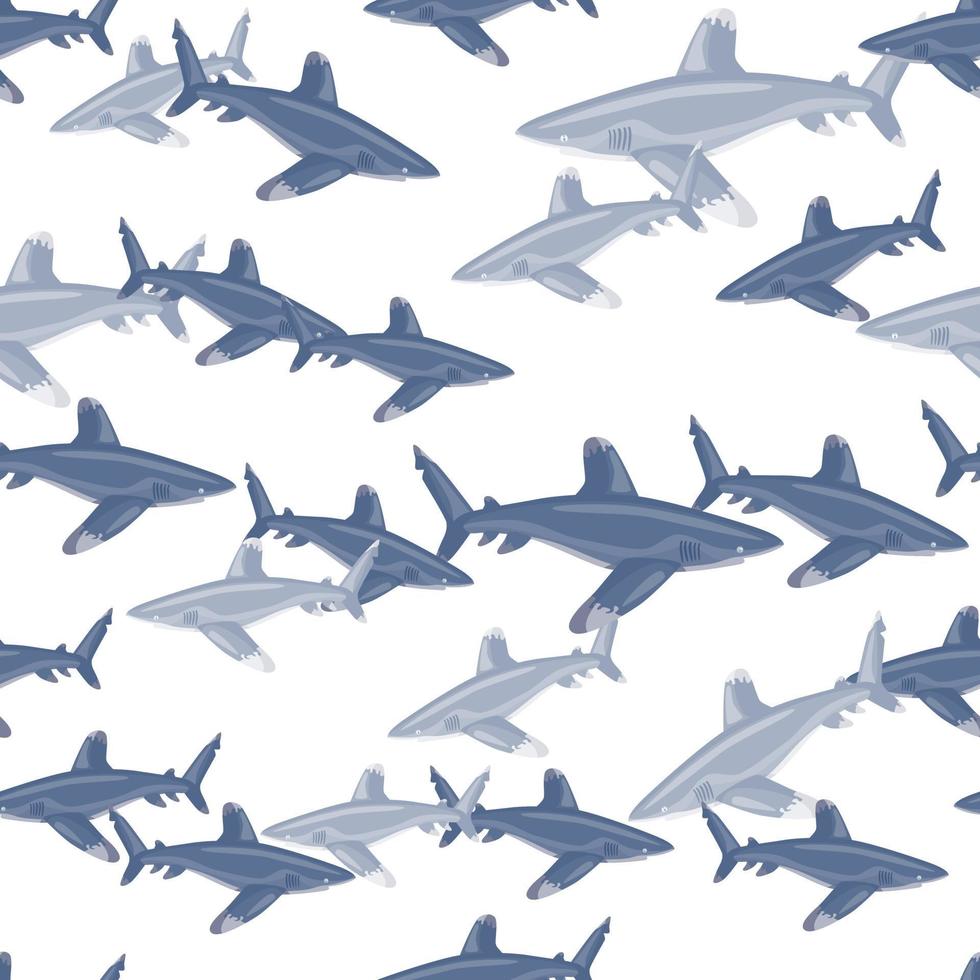This image is a computer-generated illustration featuring numerous sharks on a white background. The sharks, depicted in a simplistic, almost toy-like style with hard, unnatural lines, come in two distinct colors: light gray and dark blue-gray. The light gray sharks, all of which are swimming to the left, vary in size, with one notably large shark positioned at the top right of the image. The dark blue-gray sharks, marked by blue bodies and gray lines with rounded fins tipped in white, are primarily swimming to the right, though a few deviate from this pattern. Overall, the sharks appear to be in motion, creating a dynamic, slightly chaotic scene where some overlap and others remain separate, with a total of around 30 sharks present in the illustration.